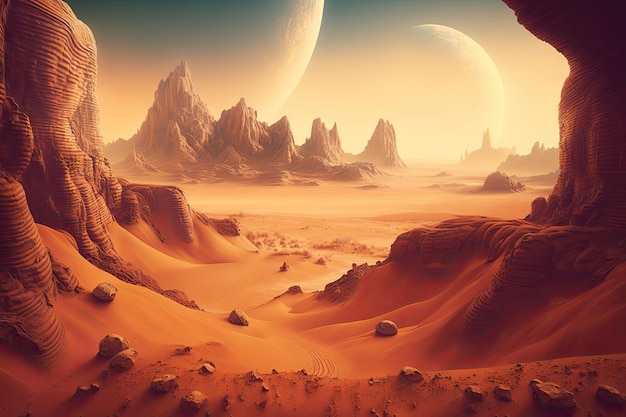This AI-generated image depicts a futuristic, alien desert landscape with striking visual elements. The scene is dominated by vast expanses of reddish-orange sand, resembling the deserts of Utah or the surface of Mars. In the foreground, smooth sand dunes stretch out, interspersed with small scattered rocks. On the left side, a towering, jagged rock formation rises dramatically, resembling a mountain. Mirroring it on the right, another large rocky structure emerges from a hill. The valley between these formations is filled with lighter orange sand and smaller rocks. 

In the distance, the landscape continues with more rugged, sharp brown stony peaks, about five in number, that punctuate the horizon. Above this, the sky transitions from a lighter hue at the horizon to a darker tone at the top, where faint outlines of two large, spherical moons or planets loom, adding an otherworldly feel to the scene. The overall palette of the image is dominated by shades of brown, orange, and yellow, with the sky exhibiting a grayish-yellow tint. The image evokes a sense of an alien world's desolate beauty, possibly reminiscent of science fiction interpretations of Mars or an exoplanet.